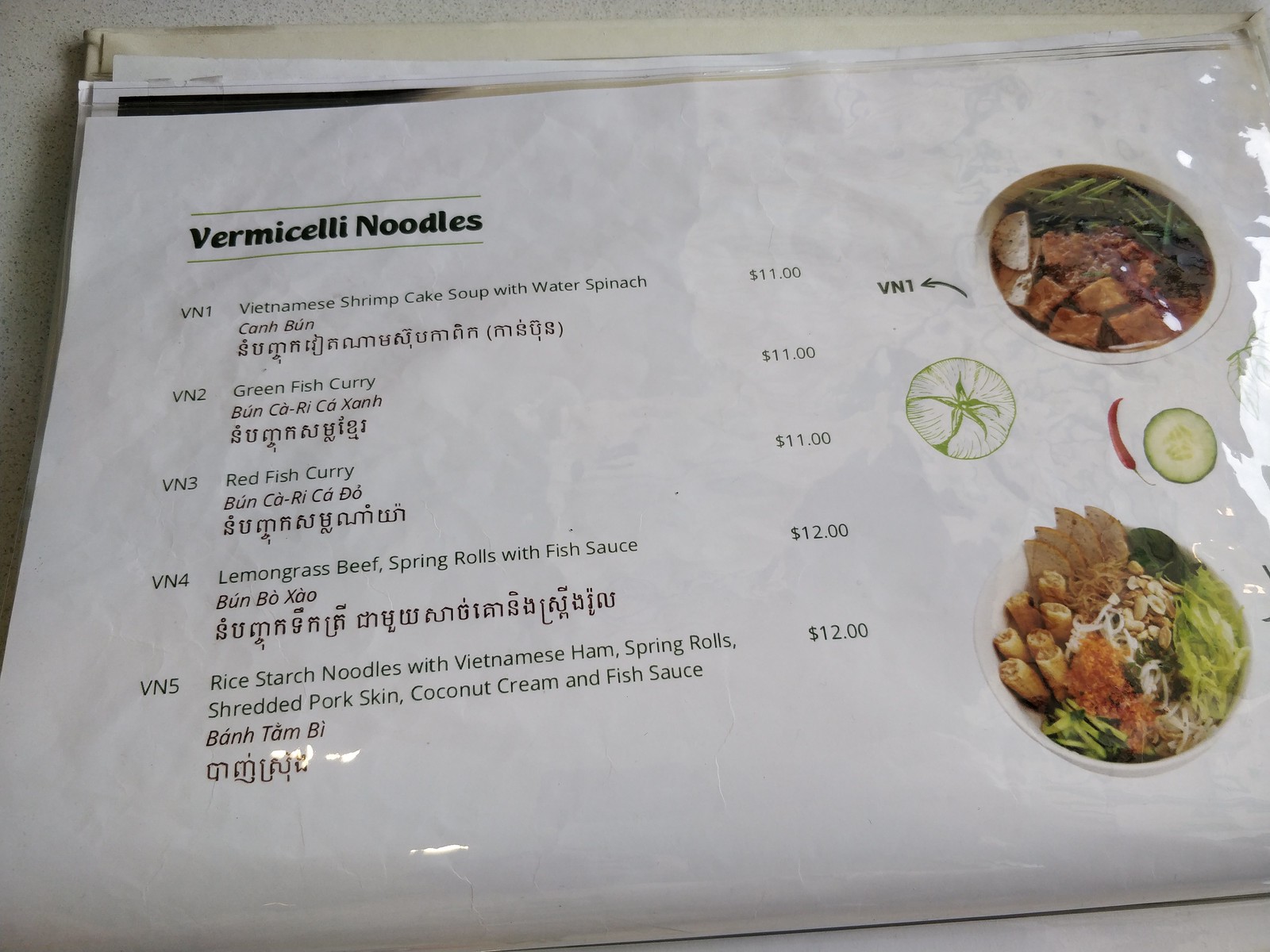The image depicts a detailed menu, focusing on the section dedicated to vermicelli noodles. The menu is white and appears to consist of multiple pages, with the current view showing a page specifically for vermicelli noodle dishes. The section title, "Vermicelli Noodles," is prominently displayed in a black font. Along the right side of the page, there are photographs of various dishes. One of these photos features a bowl of food labeled "VN1" with an arrow pointing left.

On the left side of the page, the menu details the different vermicelli noodle options available:

1. **VN1: Vietnamese Shrimp Cake Soup with Water Spinach (Canh Bún) - $11**
   - This dish features shrimp cakes served in a flavorful soup with water spinach.

2. **VN2: Green Fish Curry - $11**
   - A vibrant green fish curry, crafted with aromatic herbs and spices.

3. **VN3: Red Fish Curry - $11**
   - A rich and spicy red fish curry.

4. **VN4: Lemongrass Beef Spring Rolls with Fish Sauce - $12**
   - Spring rolls filled with savory lemongrass beef, served with a side of fish sauce.

5. **VN5: Rice Starch Noodles with Vietnamese Ham, Spring Rolls, Shredded Pork Skin, Coconut Cream, and Fish Sauce - $12**
   - A hearty combination of ingredients including Vietnamese ham, spring rolls, shredded pork skin, and a luxurious coconut cream, complemented by fish sauce.

The menu text is primarily in a lighter green color. Each dish name is presented in English, with transliterated Vietnamese and actual Vietnamese script in red. This color scheme of black, light green, and red gives the menu a vibrant yet organized appearance. 

The food images accompanying the text highlight various ingredients such as fried tofu, which appears brown, and a variety of vegetables in green. Some dishes also seem to feature an orange caviar topping. Adding to the vivid presentation are a red hot pepper and a green cucumber slice, visible on the right side of the menu.